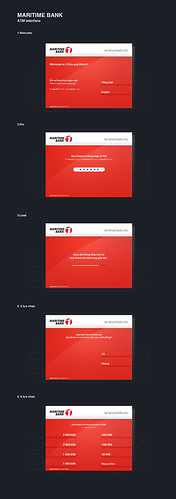The image displays a screenshot taken within the context of Maritime Bank, although it is unclear whether it is from a website or another platform as there is no header to provide that clarification. The background of the screenshot is entirely black. Positioned in the top left corner is the text "Maritime Bank" written in white. 

Dominating the center of the screenshot are five vertically aligned business cards, each primarily red with a white line banner at the top. These cards appear to be business cards associated with the Maritime Bank. However, the text on these cards is too small to be legible in the screenshot. 

Adjacent to each card on the upper left-hand corner, there is white text indicating further details or labels, but the content remains indistinguishable due to size limitations. Each card uniformly features the Maritime Bank name and logo on the upper left-hand section of the banner.